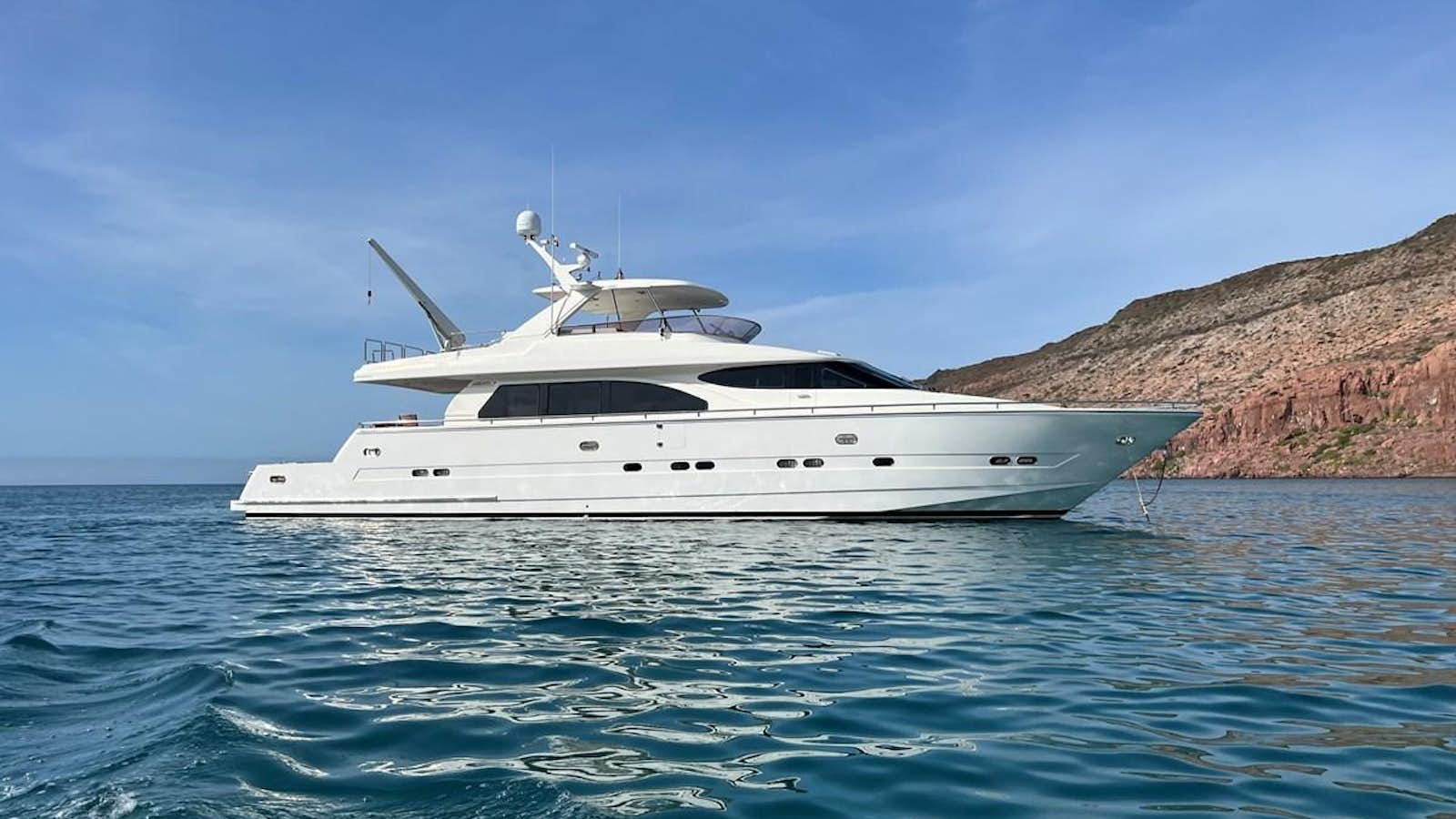The image captures a sleek white yacht centered in the middle of a picturesque landscape, occupying about half of the frame. The yacht is floating on choppy, dark blue waters, with faint reflections hinting at its presence. The vessel, appearing both fast and streamlined, features an open top displaying the steering wheel and sleek windows along its midsection. A noticeable crane or hook extends from the back, suggesting it could haul items.

Above, a mostly clear, deep blue sky with wisps of white clouds stretches halfway down the frame, meeting the horizon where water and sky converge. To the left, a sloping hill ascends, characterized by barren, brown rocky dirt interspersed with sparse vegetation or shrubs. The land behind resembles a small mountain or large hill, composed predominantly of bare rock with patches of greenery. The scene, devoid of people, emphasizes the solitary yacht in a serene yet slightly rugged setting.